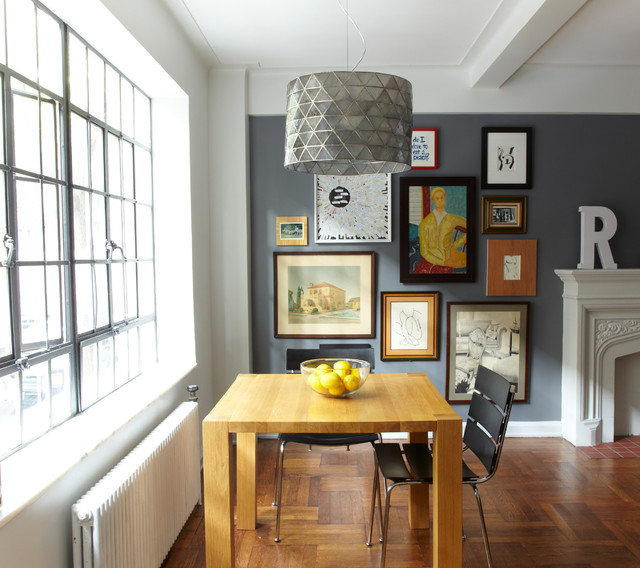This image depicts a dining room within a house that has a contemporary, warehouse-style aesthetic. On the left side, there is a large window adorned with black bars, divided into multiple rectangular panes, and equipped with a latch. A wall heater or radiator runs along the bottom underneath the window. In front of the window, there is a medium brown wooden table, holding a glass bowl filled with about six or seven lemons. Accompanying the table are two black, four-legged chairs without arms, featuring chrome details.

Suspended above the table is a futuristic-looking gray cylindrical light fixture. The back wall is painted gray and decorated with a variety of art pieces in different sizes, one of which includes an image of a man in a yellow jacket. To the right of the art cluster, there is a white fireplace, topped with a large decorative letter "R." The ceiling is white and includes a visible beam, and the flooring throughout the room is dark brown hardwood.